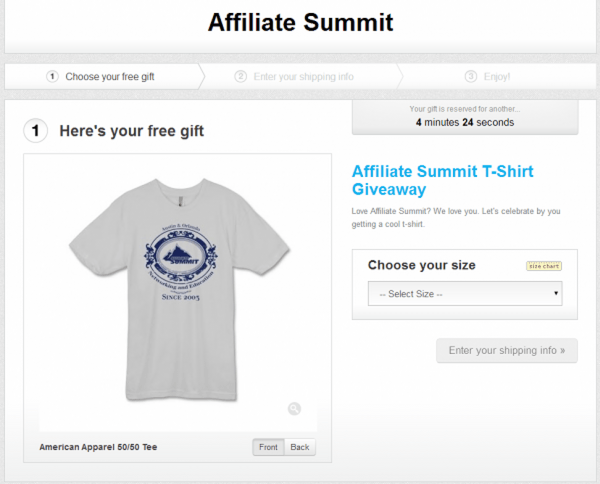***Product Page - High-Quality Merchandise Selection***

*Affiliate Summit Shopping Cart Interface*

Welcome to the Affiliate Summit merchandise page, designed for a seamless shopping experience with a clean and minimalist layout. The page features a crisp white background accented with subtle grey borders and functional buttons for navigation.

**Header:**

At the very top, the header proudly displays "Affiliate Summit" ensuring you are on the official merchandise page.

**Process Outline:**

Beneath the header, a horizontal grey border delineates three essential stages of the purchasing process:

1. **Choose Your Free Gift**
2. **Enter Your Shipping Info**
3. **Enjoy Your Gift**

**Timed Offer:**

Immediately below, another grey border emphasizes that the gift is reserved for a limited period, urging timely checkout.

**Product Display:**

1. A prominent section labeled with a large "1" introduces the gift – an "American Apparel 50/50 T-shirt."
2. The T-shirt is visually displayed in an appealing grey color, with interactive buttons allowing you to view both the front and back.

**Product Description:**

On the right side, a detailed description provides information about the T-shirt, highlighting its quality and material (50% Cotton, 50% Polyester).

**Size Selection:**

A bordered section includes:
- A button for choosing your size
- An additional button to access the size chart for precise measurements

**Checkout Button:**

At the bottom of the page, a navigation button is available for you to enter your shipping information, which will then guide you to the next step in the process.

**Conclusion:**

This straightforward and efficient layout ensures a smooth shopping experience, allowing you to easily select your free gift, enter the necessary details, and enjoy your Affiliate Summit merchandise swiftly.